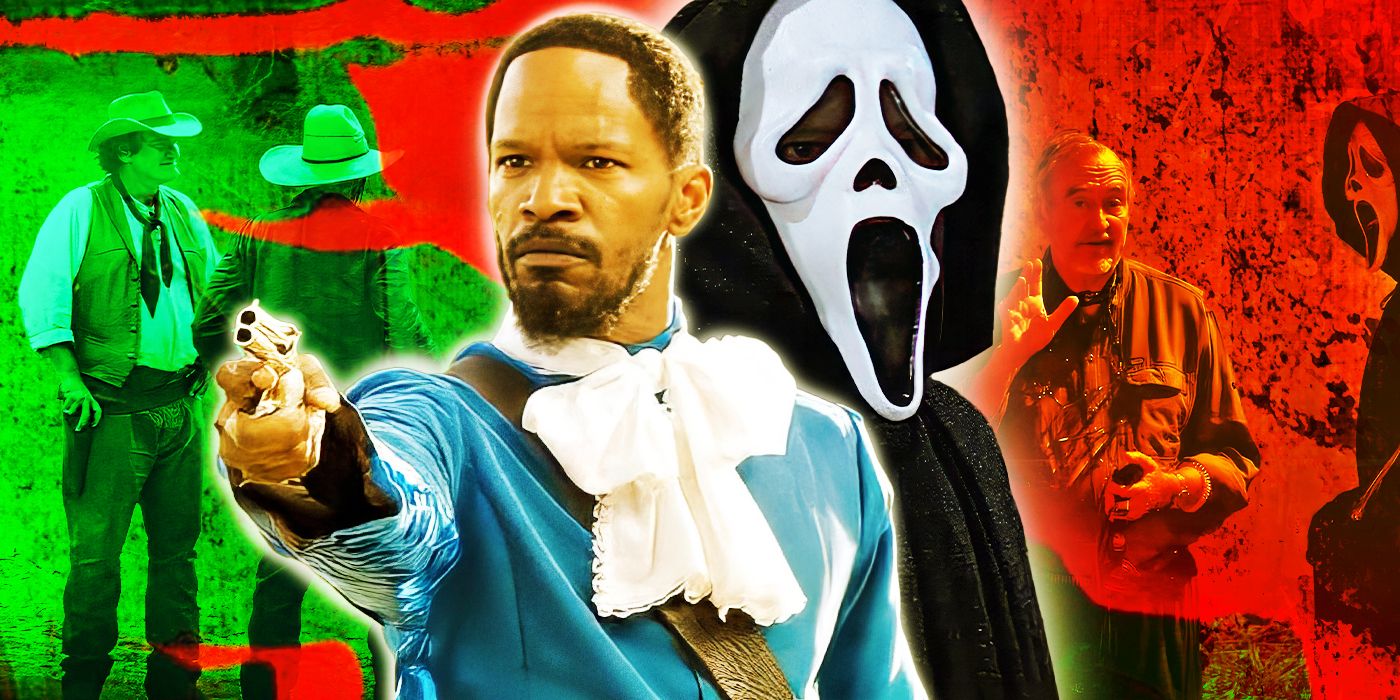This vibrant, collage-like color photo seems to blend different scenes from various movies. Dominating the central third of the image is actor Jamie Foxx, dressed in a formal blue vest adorned with a striking white bow tie, extending his right arm to point a small silver double-barrel handgun toward the viewer. Foxx wears a look of intense seriousness. Directly adjacent to him is the ominous figure of the Scream character, with its iconic white skeleton mask adding a haunting touch. The left section of the image features a green-hued scene where two men dressed as cowboys, with hats, bow ties, and vests, appear to be conversing in a field. On the opposite side, the right section is primarily red and depicts a man, possibly a director, raising his hand as if instructing someone, with another appearance of the Scream character lurking menacingly behind him. The backdrop includes splashes of color, enhancing the eclectic, intense atmosphere of the composition.